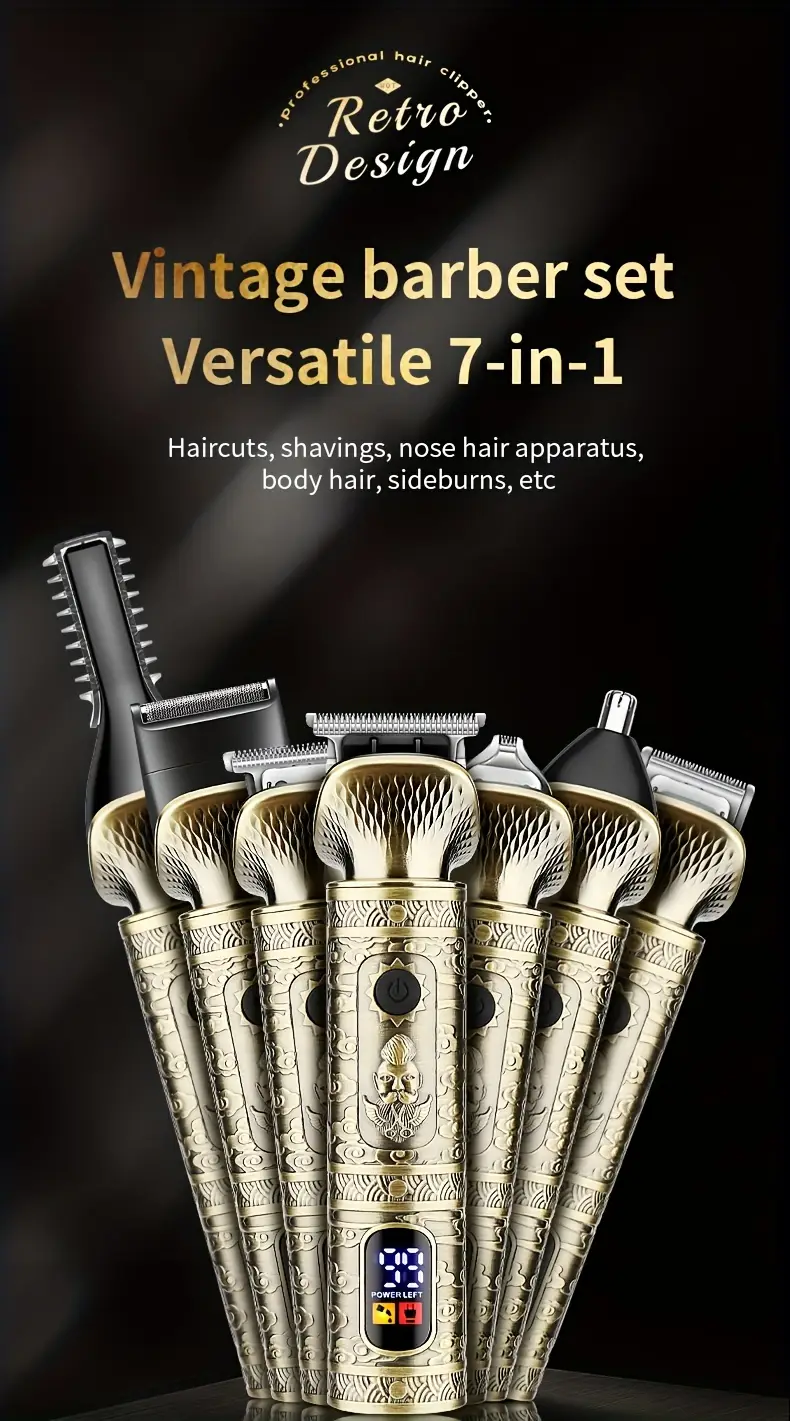The advertisement features a vintage barber set, highlighted as a versatile 7-in-1 tool for haircuts, shavings, nose hair maintenance, body hair trimming, and sideburns. Set against a black background adorned with faint diagonal light rays, the layout is centered around chrome-plated tools fanned out elegantly. The tools, which include clippers, a comb, a razor, and scissors, boast a retro-futuristic design with intricate golden engravings. Prominently, the upper part of the ad displays the title "Professional Hair" in an ornate font, with "Retro Design Clippers" in a blockier typeface just below. Additional text in white and gold reinforces the multifunctionality of the set. The logo "99 Powerlift" is also visible, enhancing the ad's vintage yet sophisticated aesthetic.